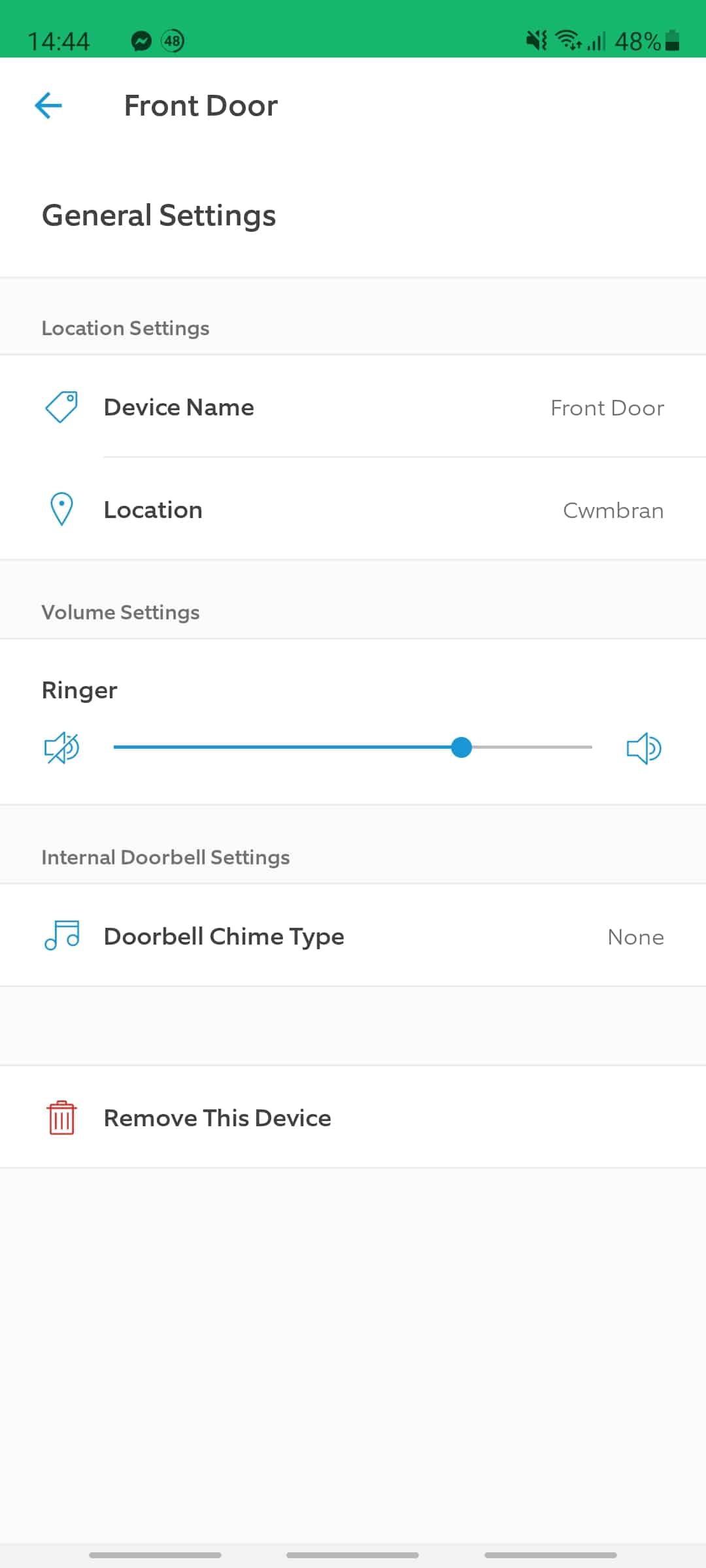The image depicts a close-up view of a smartphone screen displaying the settings for a front door device. The phone is at 48% battery life and the time is 14:44 in military format. A blue back arrow is visible on the top left, labeled "Front Door," indicating you can return to the previous menu. Under the "General Settings" section, various options are listed: 

1. **Location Settings**: The location is pinned to CWMBRAN.
2. **Device Name**: Displayed as "Front Door" with an icon beside it.
3. **Volume Settings**: The ringer volume is adjustable from completely silent to very loud and is currently set to about three-quarters of the maximum level.
4. **Internal Doorbell Settings**: Includes options for door chime types, but currently, no internal doorbell chime is selected.

At the bottom, there's an option to remove the device, represented by a picture of a garbage can. Additionally, there's a gray box for making notes, accompanied by three vertical gray lines at the bottom of the screen.